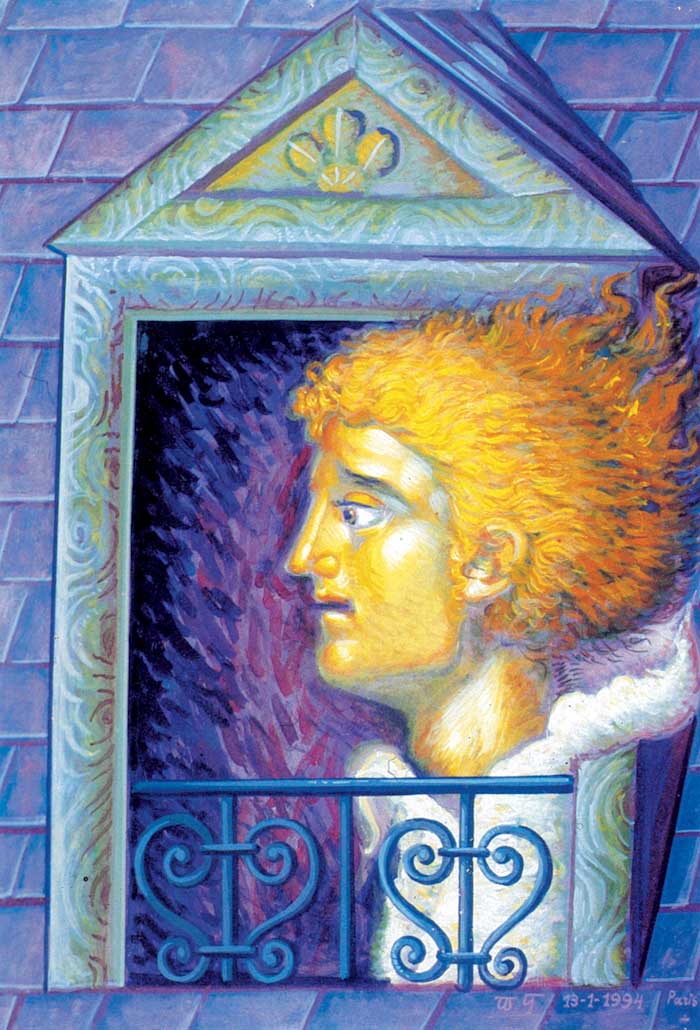This is a detailed painting depicting the side profile of a person’s head emerging from a window of a house, with only the face, neck, and part of the shoulders visible. The person’s face is painted in light brown and yellow shades, with hair in hues of yellow and orange, styled to mimic the shape of flames. The expression on the person’s face conveys slight distress as they look toward the left. The head appears to be adorned in what seems to be a white attire.

The window frame is composed of a mix of green, yellow, and grey colors, surrounding a dark interior painted in black and purple tones. The brick wall outside the window is blue. Additionally, blue railings are visible in front of the window. Above the window, there is a triangular section embellished with yellow, blue, and lighter blue colors and a central four-petal yellow flower with white lines.

The house’s roof is depicted with shingles in an array of blue, purple, and greyish tones, with a portion extending around the window. The overall color scheme of the room and the roof blends purples and blues. The bottom right corner of the painting features a date, 13-1-1994, and the word “Paris,” both written in purple, along with an artist’s signature resembling "WY" with lines over it.